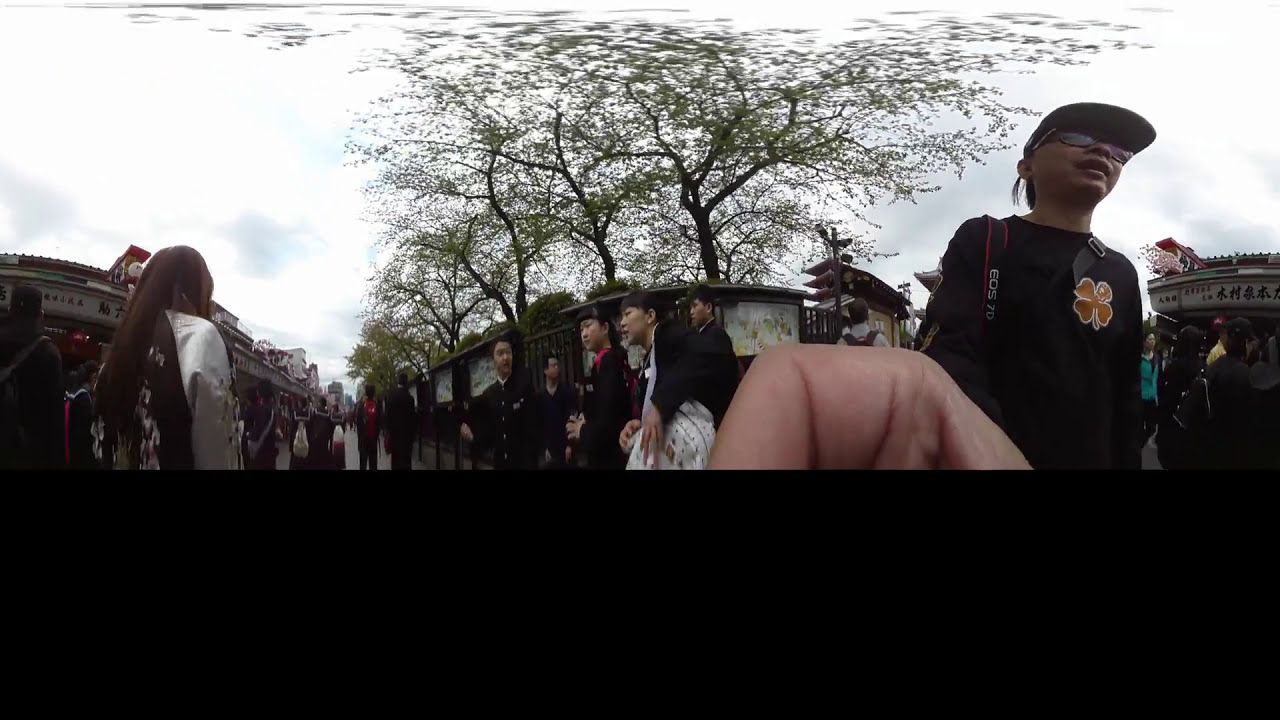This panoramic image captures a bustling crowd in what appears to be a chilly outdoor setting, possibly in a Southeast Asian country. The sky is overcast and gray, adding to the cool atmosphere. In the foreground, there's a young man in a long-sleeved black shirt adorned with a gold four-leaf clover. He wears a baseball cap and glasses, and a strap—likely from a book bag—rests on his shoulder. His body faces the viewer while his gaze is directed slightly upwards and to the right. 

On the right side of the picture, near the bottom, a distorted finger curiously juts into the frame. The scene is set in a narrow walkway bordered by buildings on the left and placards or informational signs on the right. A group of people, all dressed in dark outfits and some wearing jackets, fills the walkway. In the background, there seem to be two main structures; one resembling a train and another potentially a carnival booth or food stand. Leafless trees surge towards the top of the image, framing the outdoor venue where the crowd appears to be waiting or gathering.